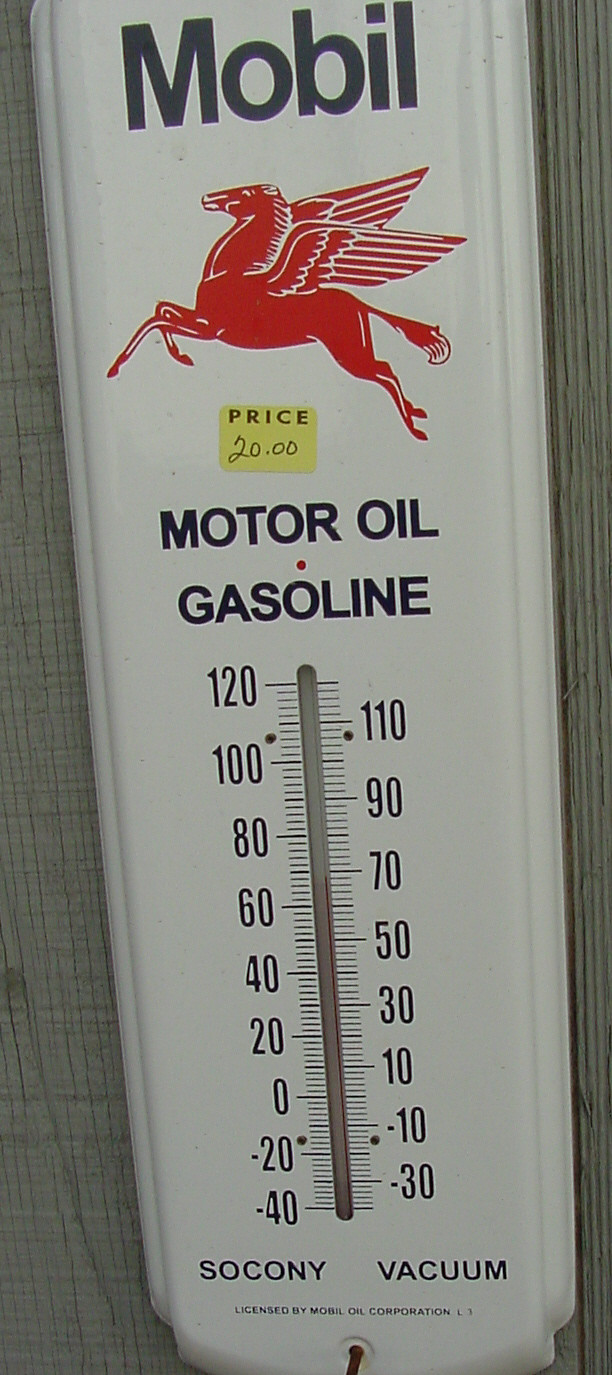The close-up photograph captures a vintage outdoor thermometer attached to the exterior of a weathered wooden building. The building's wood appears aged and gray, enhancing the rustic charm of the scene. The thermometer itself is crafted from metal and painted white, featuring the branding "MOBIL" in bold black letters at the top. Just below the brand name, a vivid red winged horse, symbolic of Mobil's Pegasus logo, seems to be in flight. Affixed to the thermometer is a small yellow tag with the word "price" and a handwritten $20 note. Further down, the inscriptions "motor oil" and "gasoline" are displayed in black text. The thermometer scale ranges from 0 to 120 degrees Fahrenheit, with the current temperature reading around 68 or 69 degrees. At the very bottom, the terms "SOCONY" and "VACUUM" are printed, alluding to the historical companies associated with the Mobil brand. The entire composition exudes a nostalgic, bygone era.